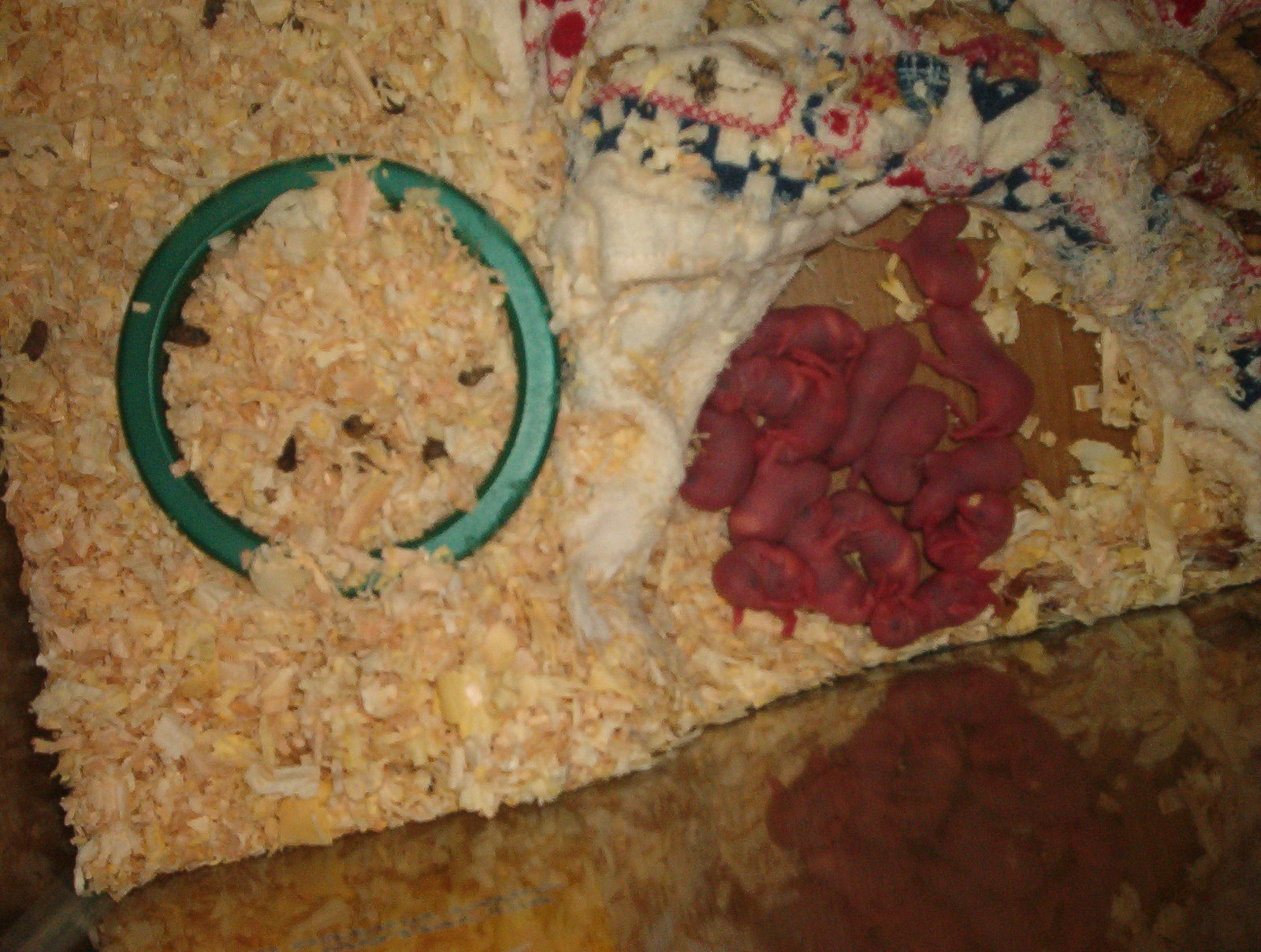This image shows a top-down perspective of what appears to be an old aquarium repurposed as a hamster or rodent cage. The cage contains pale wood chip bedding and a green dish filled with shavings. Scattered across the bedding are rodent droppings. On the right side of the image, there are approximately 10 to 20 newborn rodents, possibly baby hamsters, mice, or rats. These tiny creatures are a striking, dark red color, indicating their very recent birth. Surrounding the newly born rodents are signs of nesting, including an old, shredded kitchen towel that features a mix of white, blue, and red threads. The rodents are huddled together in a circle, lying on and next to each other, giving a clear view of their undeveloped, fur-less skin. The background of the cage includes some scattered, yellow and beige feed scraps, possibly meant as food for the animals.